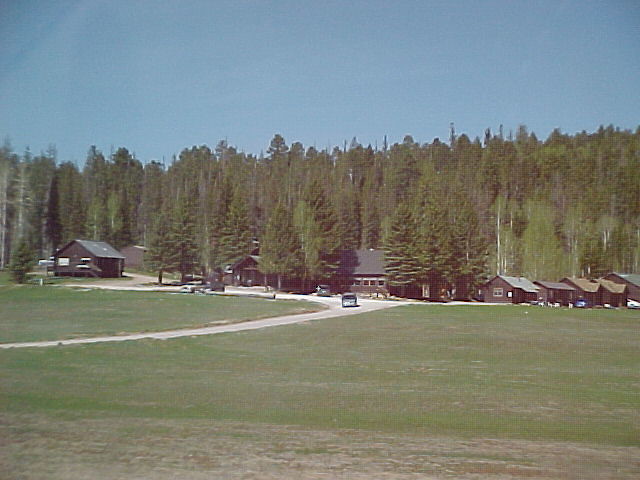The photograph captures a picturesque log cabin campground nestled in a lush, forested landscape. The scene is set on a clear, sunny day, with vibrant green grass and an abundance of tall pine trees, some of which have bare branches. The lower left-hand side of the image features a dirt road that curves to the right and extends into the distance, intersecting a network of cabin-lined paths. The campground comprises several log cabins, each characterized by their brown timber construction and some adorned with wooden steps. A blue car and a white car are visible, illustrating the active presence of visitors. Beyond the cabins and the road, the terrain appears to gently rise, giving way to a dense forest that stretches up the hills in the background. This serene setting evokes an ideal place for relaxation and vacation, surrounded by nature's tranquility.